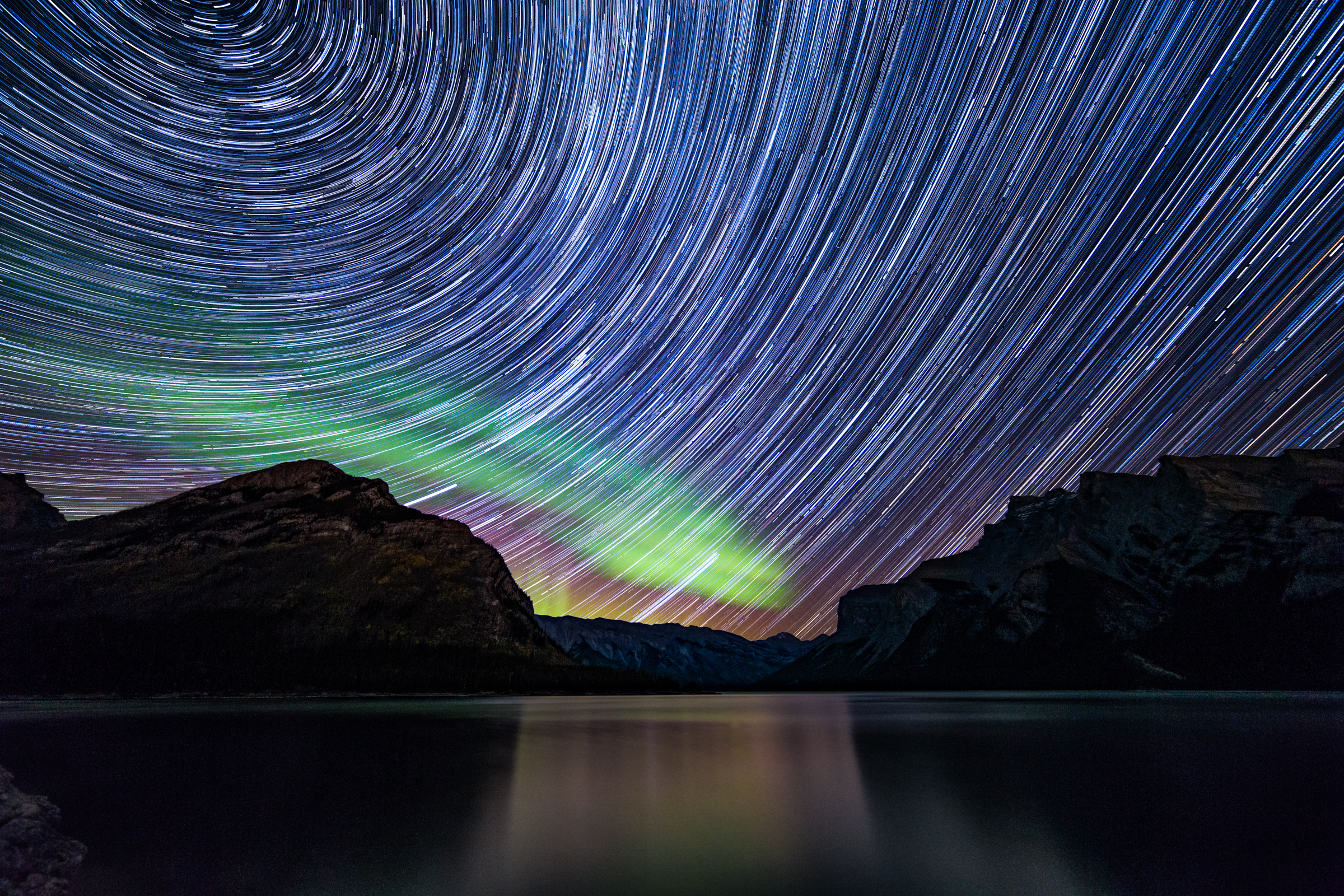A mesmerizing and surreal time-lapse photo captures the aurora borealis illuminating the night sky over an expansive, smooth lake, against a backdrop of rugged, craggy mountains likely situated in a northern region such as Iceland, Greenland, or Alaska. The sky, predominantly in hues of bluish-purple with traces of green, pink, yellow, orange, and red, showcases a striking array of circular white designs and dynamic, colorful lines, creating an intricate web that spirals around a central vortex point, a hallmark of polar photography. This ethereal display reflects off the lighter central axis of the lake, enhancing the otherworldly atmosphere, while the vivid ribbons formed by the time-lapsed stars draw intricate, impossible patterns that contrast with the natural beauty of the aurora borealis above the rocky horizon.